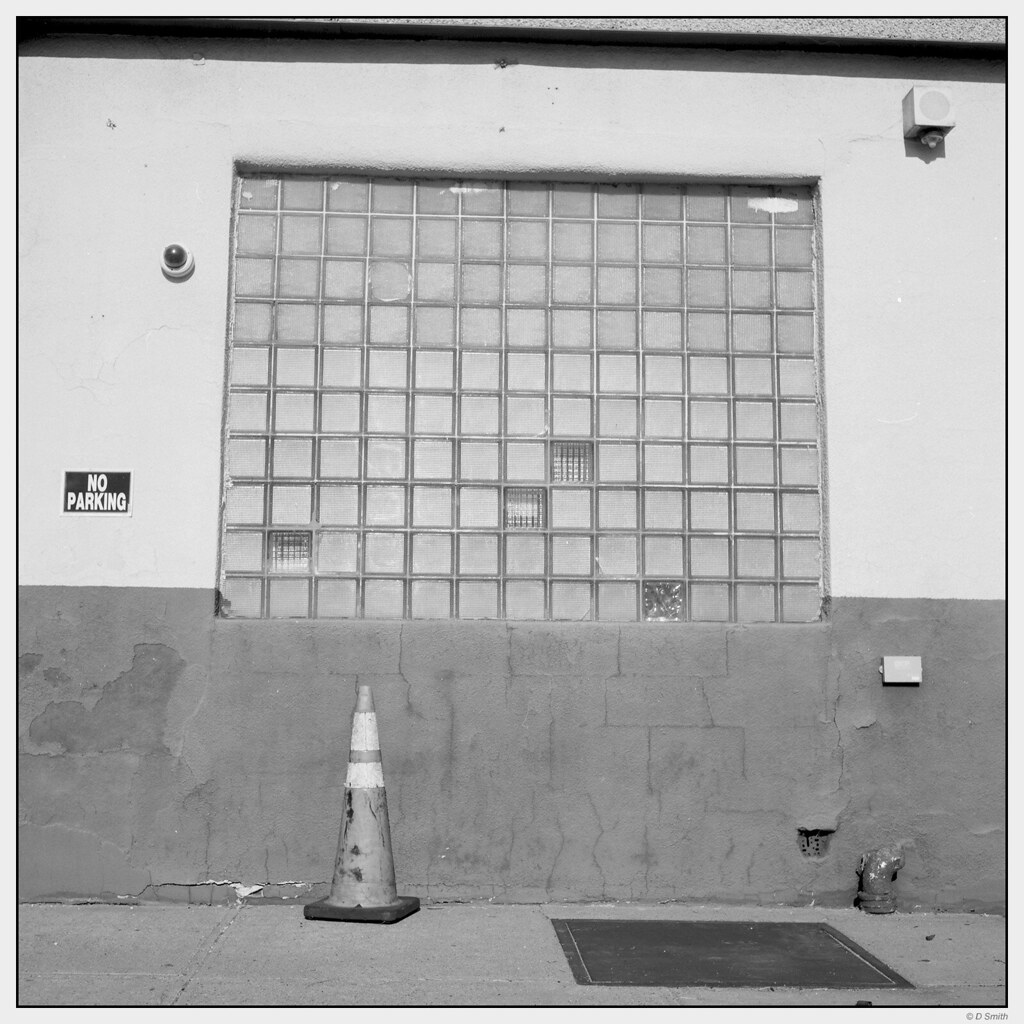The exterior of an old building is captured in this black and white photograph. The building features a large central window composed of about 100 small, frosted glass squares, arranged in a grid, reminiscent of a checkerboard pattern. This window, which allows light to enter while obscuring visibility, dominates the middle of the photograph. To the left of the window, a "No Parking" sign is affixed to the wall, with a circular 360-degree security camera positioned above it. On the right side of the window, near the top, there appears to be a speaker or alarm box. The lower part of the building's exterior wall is painted a dark color, transitioning to white a few feet above the ground. In the foreground, a metal grate or hatch is set into the sidewalk next to a hole that appears to lead underground. A caution cone, likely orange with two white stripes, stands nearby, slightly to the left of the window, adding an element of safety to the scene. Additionally, a small pipe emerges from the building near the bottom right corner of the photograph.